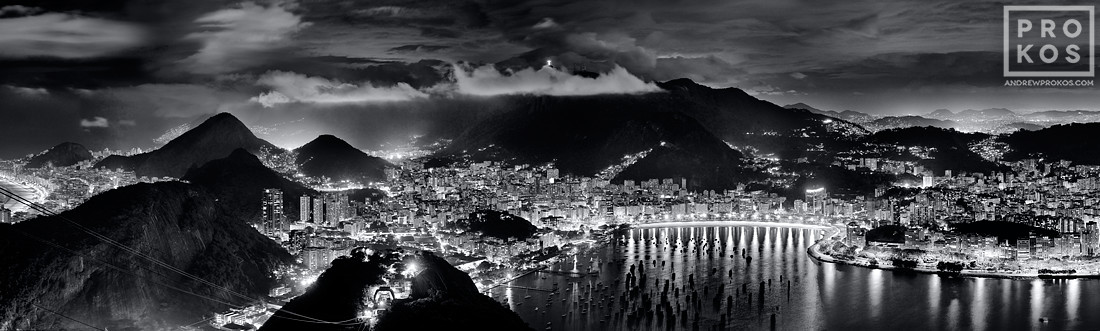This black and white photograph captures a striking cityscape at night, dominated by the sharp contrast of illuminated buildings and the dark skyline. In the top right corner, a watermark reads "Prokos" with the website "andrewprokos.com," identifying the creator. The city is nestled against towering mountains, with winding streets and potential waterways – although the absence of color makes it difficult to discern whether it is water or possibly an ice-skating ring. The scene is further animated by clouds and a vast sky. The bright city lights from homes and buildings highlight the city’s density and vibrancy, while power lines add to the urban feel. This 16x9 horizontal photograph offers a comprehensive view of a bustling, populous city seamlessly integrated into its natural mountainous surroundings.